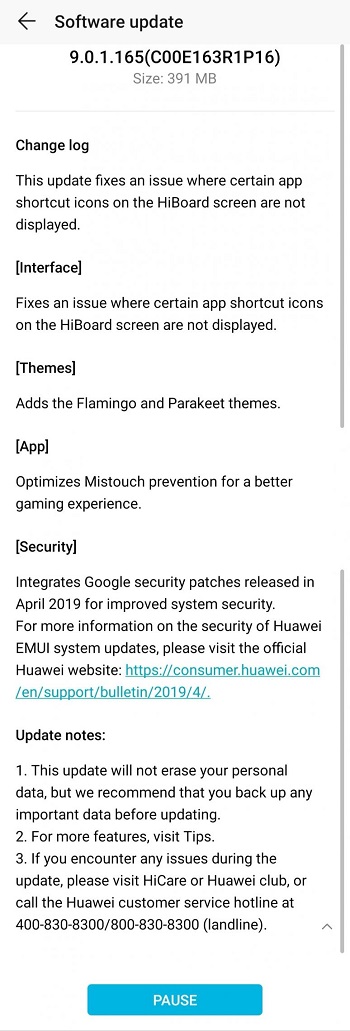This image is a screenshot captured from a Huawei mobile device, displayed with a light background. The screenshot showcases the 'Settings' menu specifically under the 'Software Update' section. 

At the top of the screen, a gray banner contains the heading "Software Update." Directly below this, the software version "9.0.1.165" is prominently featured, followed by a series of alphanumeric codes enclosed in parentheses. The size of the update is listed as "391 megabytes."

The screen proceeds to outline the 'Change Log,' detailing several updates and fixes:
1. **Fixes an issue where certain app shortcut icons on the high board screen are not displayed.**
2. **Interface:** Addresses the same issue with app shortcut icons on the high board screen.
3. **Themes:** Introduces two new themes named "Flamingo" and "Parakeet."
4. **App:** Enhances mis-touch prevention to improve the gaming experience.
5. **Security:** Includes unspecified security-related updates.

At the bottom, under the 'Update Notes' section, three distinct notes are presented sequentially. Finally, a prominent blue button labeled "Pause" in white text is located at the bottom of the screen.

Overall, this detailed screenshot captures the essence of a typical software update menu on a Huawei Android device, highlighting new features, fixes, and enhancements.